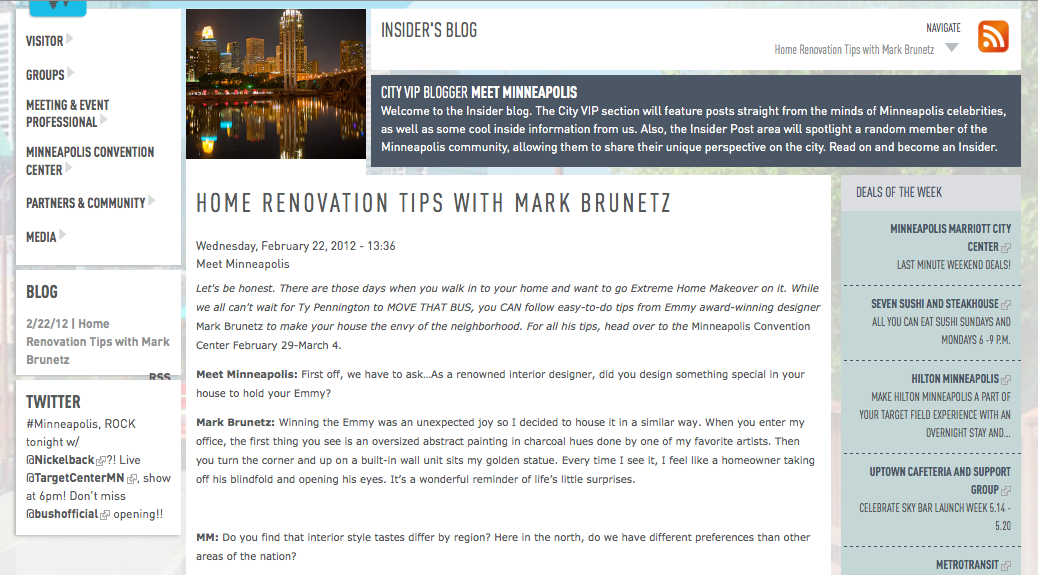This desktop screenshot provides a detailed view of the "Insider's Blog" homepage. Positioned prominently at the top-center is the blog's title, "Insider's Blog," accompanied by a "Navigate" drop-down menu to the right.

Below this, a feature description titled "Home Renovation Tips with Mark Brunettes" is visible, to the right of which is an orange square icon depicting a diagonally positioned Wi-Fi signal.

The center section below "Insider's Blog" introduces the City's VIP Blogger section with the title "Meet Minneapolis." A warm welcome is extended, explaining that this section will highlight posts from Minneapolis celebrities and offer insider information. Additionally, the "Insider Post" area will spotlight random community members, allowing them to share their unique perspectives on the city, inviting readers to "Read on and become an insider."

To the left of this text is a stunning image of the night skyline of Minneapolis, framed by several clickable buttons with right-facing grayed-out arrows. These buttons lead to various sections such as "Visitor," "Groups," "Meeting and Event Professionals," "Minneapolis Convention Center," "Partners and Community," and "Media."

Below this section, a separate white square is dedicated to blog updates marked simply as "Blog," and yet another square underneath it connects to Twitter, featuring hashtags like #MinneapolisRock, #TonightWithNickelbackLive, #TargetCenter, #Minnesota, #MN, "Show at 6 PM," "Don't Miss," concluding with "@BushOfficialOpening."

In the middle and predominantly composed of a white background, further details about "Home Renovation Tips with Mark Brunettes" are found. A timestamp reads Wednesday, February 22, 2012, at 13:36. It invites readers to meet Mark Brunettes and includes a short teaser: "Let's be honest, there are those days when you walk into your home and want to go extreme home makeover on it. While we all can't wait for Ty Pennington to move that bus, you can follow easy-to-do tips from Emmy Award-winning designer, Mark Brunettes, to make your house the envy of the neighborhood." For those interested in more tips, it directs them to the Minneapolis Convention Center event, taking place from February 29 to March 4.